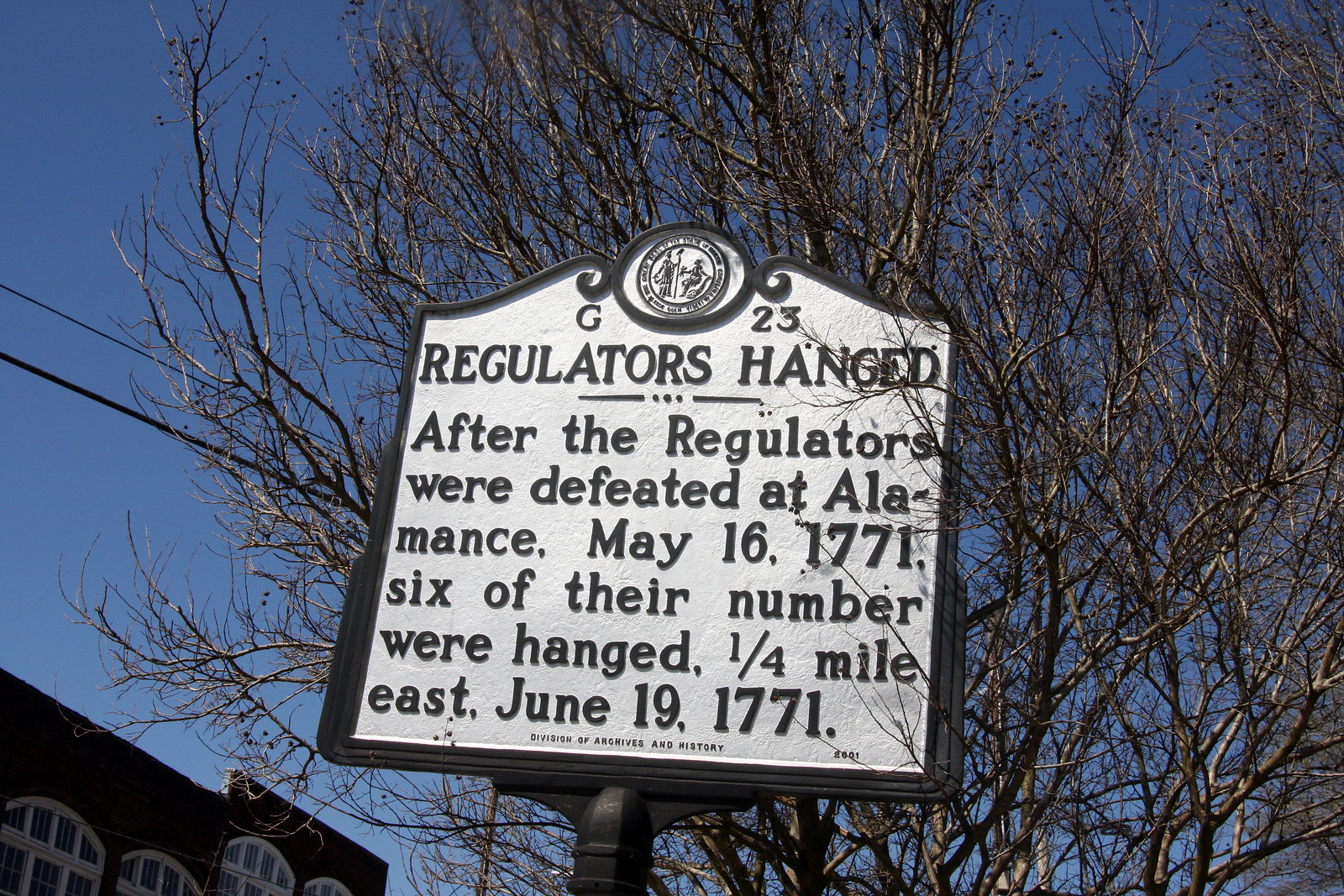The photograph features a prominently displayed metal sign with a white background and a black border. The sign has a distinct beveled, rounded top with an emblem situated at the uppermost portion. On either side of the emblem, it is marked with the symbols "G" on the left and "23" on the right. The sign bears black-etched text detailing a historical event: "Regulators hanged. After the Regulators were defeated at Alamance, May 16, 1771, six of their number were hanged a quarter mile east, June 19, 1771." 

The surrounding environment depicted in the photograph includes a leafless tree, indicative of a winter setting, with its bare branches extending against a clear blue sky. To the left of the sign, there's a portion of an older building featuring curved windows and adjacent to it, a visible power line. This setting suggests a historical area, providing context to the memorial's significance.